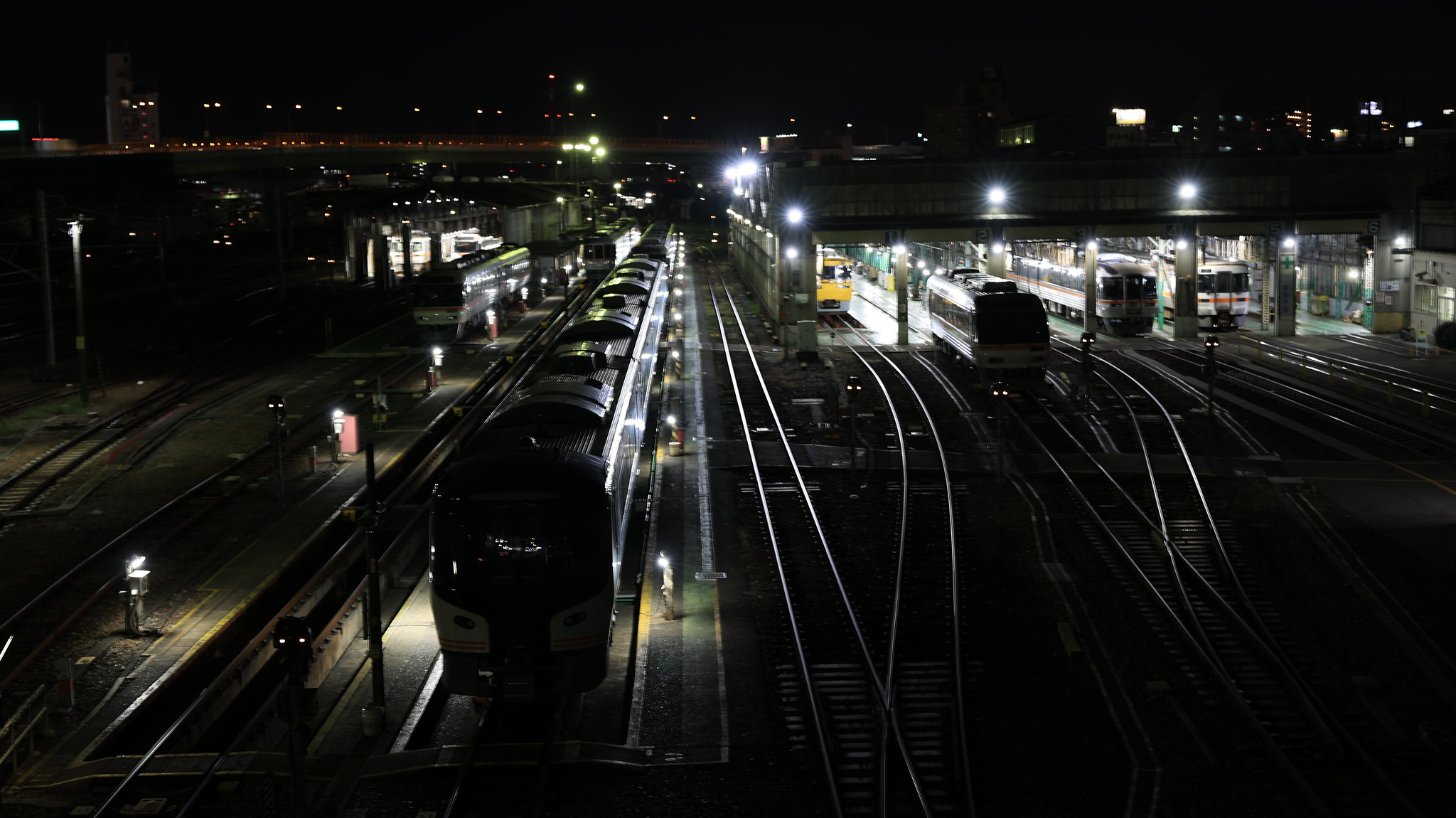This nighttime photograph captures a bustling railway station or train yard illuminated by various bright lights. The scene features seven distinct trains positioned on parallel tracks, some of which curve slightly. Two of the trains appear to be white, and one is clearly visible in yellow. The remaining trains are less discernible due to the darkness. The image includes a depot area situated in the top right quadrant. In the distant background, the lights of a distant city, including buildings and signs, can be made out. The station seems to be in operation despite the absence of people, indicated by the illuminated surroundings, including a combination of sodium and wall pack lights.